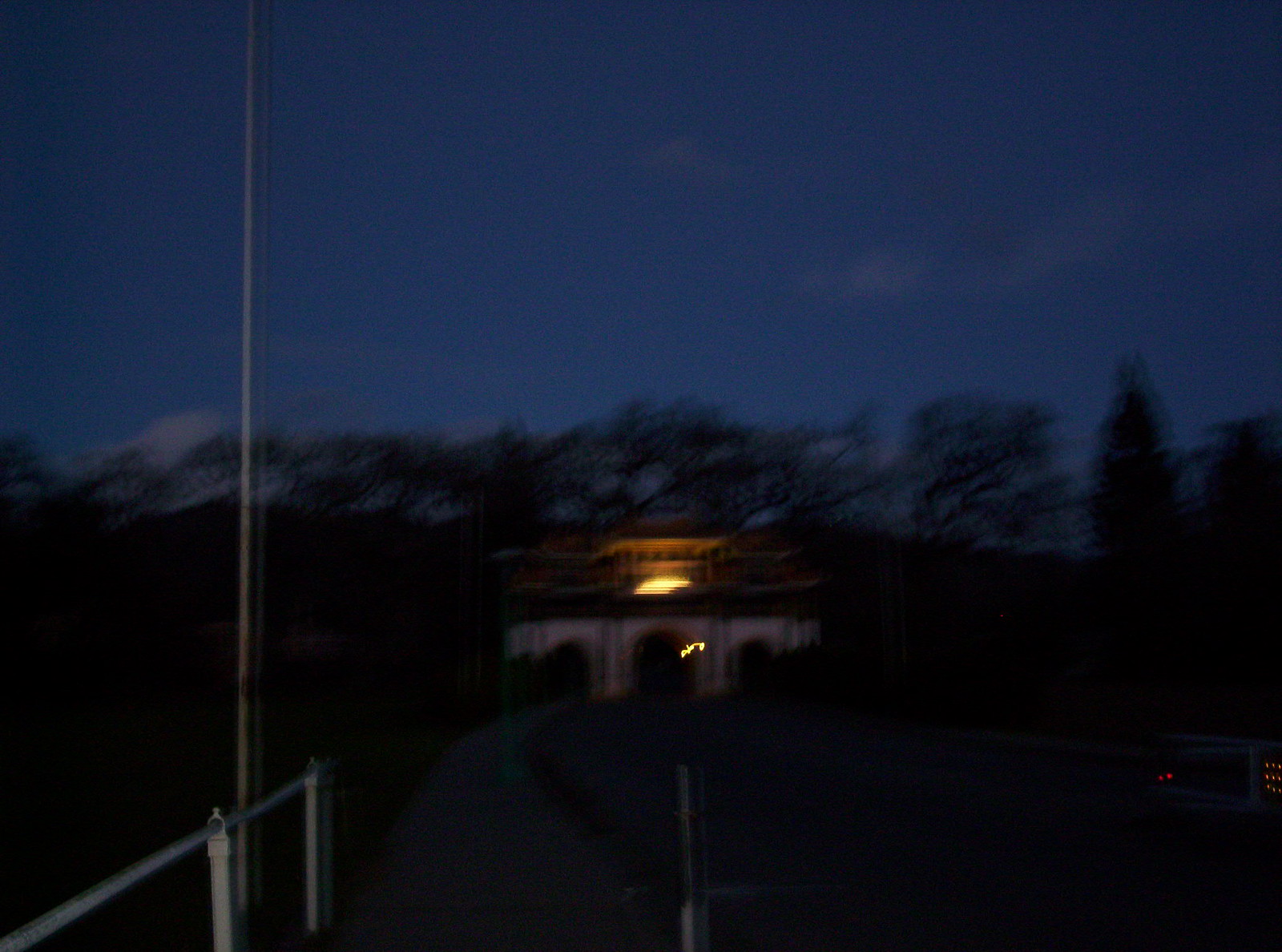Captured in the mystique of the night, the photograph reveals a blurry yet intriguing scene dominated by a two-story structure with a bright light on the upper level. The building, possibly resembling a coliseum or a grand house, features multiple arches on its lower floor, creating an air of extravagance despite the low visibility. The dark, royal blue sky with faint, faded gray clouds hints at the cusp of deepest night. Centered within the frame, the building stands atop a hill, accessible by a road with a dividing line, suggesting the photographer aimed straight down this path. Surrounding the edifice is a line of dark, indistinct trees forming a shadowy background. On the left side of the image, near the photographer, there seems to be a railing or possibly a stairwell, and behind it, a faint outline of fencing is visible. The overall atmosphere is dark and blurred, contributing to the enigmatic and somewhat eerie quality of the scene.